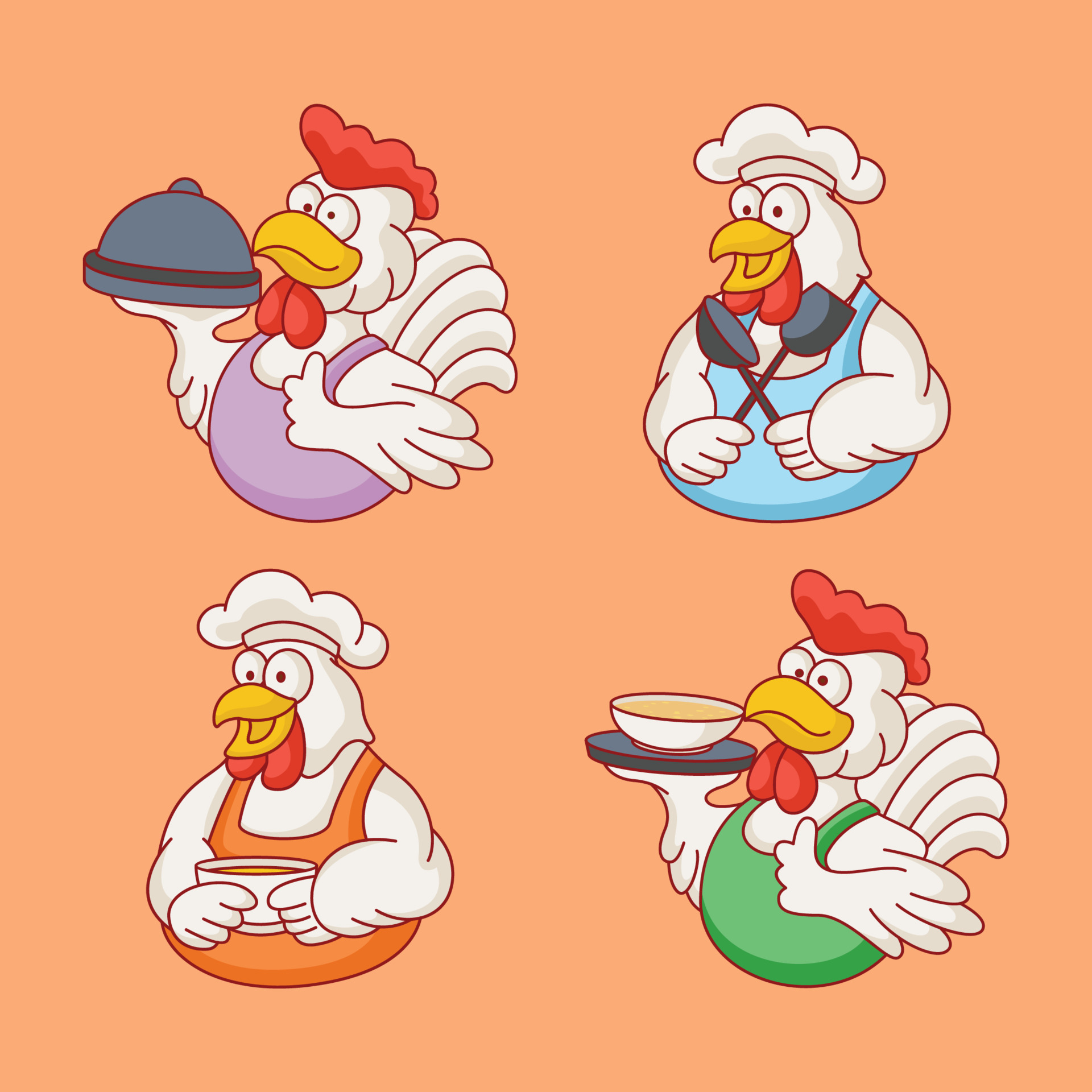This is a cartoon illustration featuring four white chickens with yellow beaks and red wattles, giving the appearance of neckties. The background is a light orange, almost salmon color, and the chickens are arranged in a square. Each chicken is dressed in a food-themed outfit and dons a colored vest: purple, blue, green, and orange. 

- The top left chicken, wearing a purple vest and visible red comb, holds a plate covered with a warming dome in its right wing and gives a thumbs up with its left wing.
- The top right chicken sports a blue vest and a white chef's hat, holding a spatula and ladle crossed in front of it, with its beak open.
- The bottom left chicken in an orange vest also wears a white chef's hat and holds a bowl of liquid, with its beak open.
- The bottom right chicken in a green vest presents a tray with an open bowl of soup and gives a thumbs up with its left wing.

All four chickens exhibit different gestures and accessories, contributing to a whimsical culinary theme.